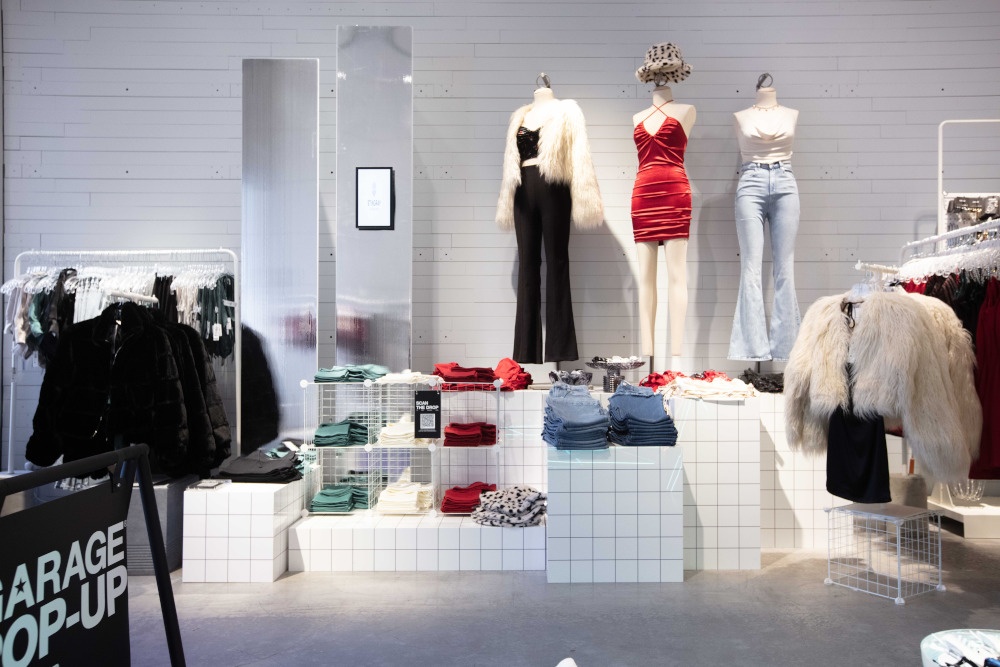This image is a detailed photograph of a closed women's clothing store with a sign in the bottom left corner reading "GARAGE POP-UP" partially cropped out. The store has gray flooring and features three mannequins displayed on a white gridded structure that doubles as a platform, with neatly folded clothes on top and for sale below. 

The mannequin on the left is dressed in black pants and a black bra top, complemented by a white faux fur jacket. The central mannequin sports a striking red, sleeveless, velvety party dress paired with a white and black faux fur hat. The rightmost mannequin showcases light-wash bell-bottom jeans and a white sleeveless top. 

To the left of the mannequins, two long mirrors face the viewer, while nearby racks display various clothing. On the right clothing rack, a white fluffy jacket is prominently featured, and beneath it, more garments are arranged on tiled platforms. The left clothing rack holds black attire, including what appears to be a black puffer jacket. The entire setting combines to create an inviting, fashionable display space.